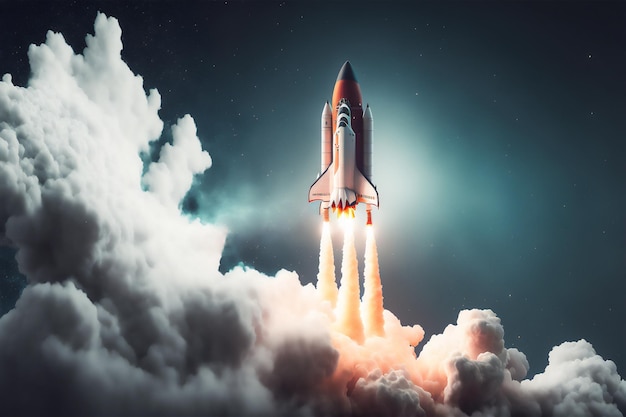This detailed image portrays a computer-rendered depiction of a space shuttle launch. The shuttle, resembling classic U.S. spacecraft like Endeavor or Challenger, is white with black accents. It's attached to a large booster rocket, which is predominantly orange with a black-tipped nose, and flanked by two smaller white rocket boosters on either side.

The scene captures the dramatic moment of liftoff, with the shuttle breaking through an L-shaped formation of clouds situated predominantly on the bottom and left. Bright yellow flames and dense plumes of white and red smoke emanate from the rocket boosters, dispersing across the ground and creating a fiery glow.

The backdrop is a dark, star-studded sky with hues of bluish-black, resembling a night sky or deep space. The stark, glowing light from either a sun or moon and a bright nebulous cloud illuminate the rocket, accentuating its ascent. Together, these elements vividly bring to life the power and awe of a rocket launching into space.